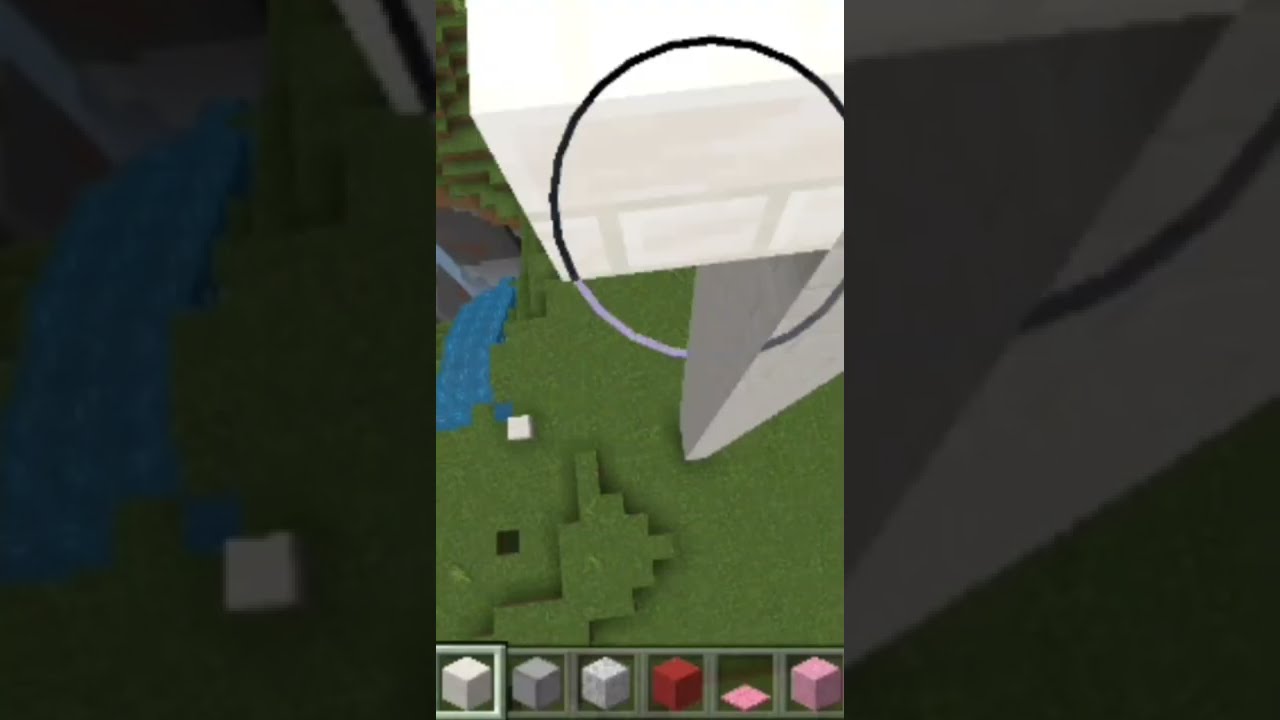The image is a composite divided into three vertical sections. The middle section showcases a screenshot from a Minecraft-style video game, presented in a bird's-eye view. Dominating the middle section is a ground area carpeted in green grass, adjacent to a white building shaped like the number seven, which features a notable circular detail. A blue river runs along the left side of this ground area. At the bottom of this section, a block selector displays an assortment of colored cubes, including various shades of gray, a red block, a no-block symbol, and a purple block. The left and right sections of the image are darkened close-ups of the respective corresponding parts from the central section, emphasizing the pixelated environment and details of the game's interface.